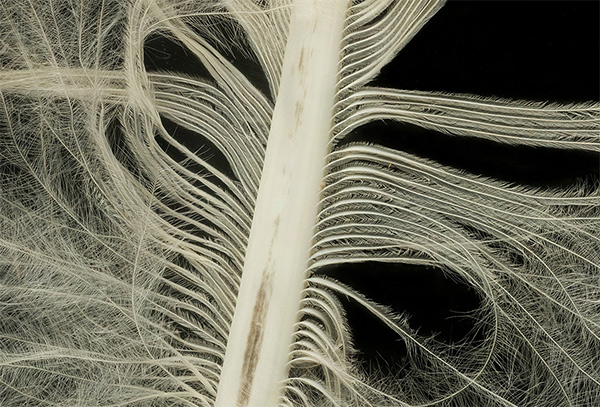This is a detailed black-and-white macro photograph that captures a close-up section of a feather. At the center of the image is a white stem, running vertically from the bottom middle to the top middle. The feather's barbs branch out from this central stem, appearing as tiny, wispy plumes. The left side of the feather is densely packed, appearing lush and thick, with the barbs closely condensed. In contrast, the right side is sparser, with some barbs seemingly missing, creating noticeable gaps. The barbs on both sides are delicate and light, contributing to the feather's intricate, airy structure. The entire composition is set against a stark black background, highlighting the feather's off-white, creamy hue. The photograph's macro lens magnification provides an intimate view, emphasizing the fine details of the feather's unique structure.